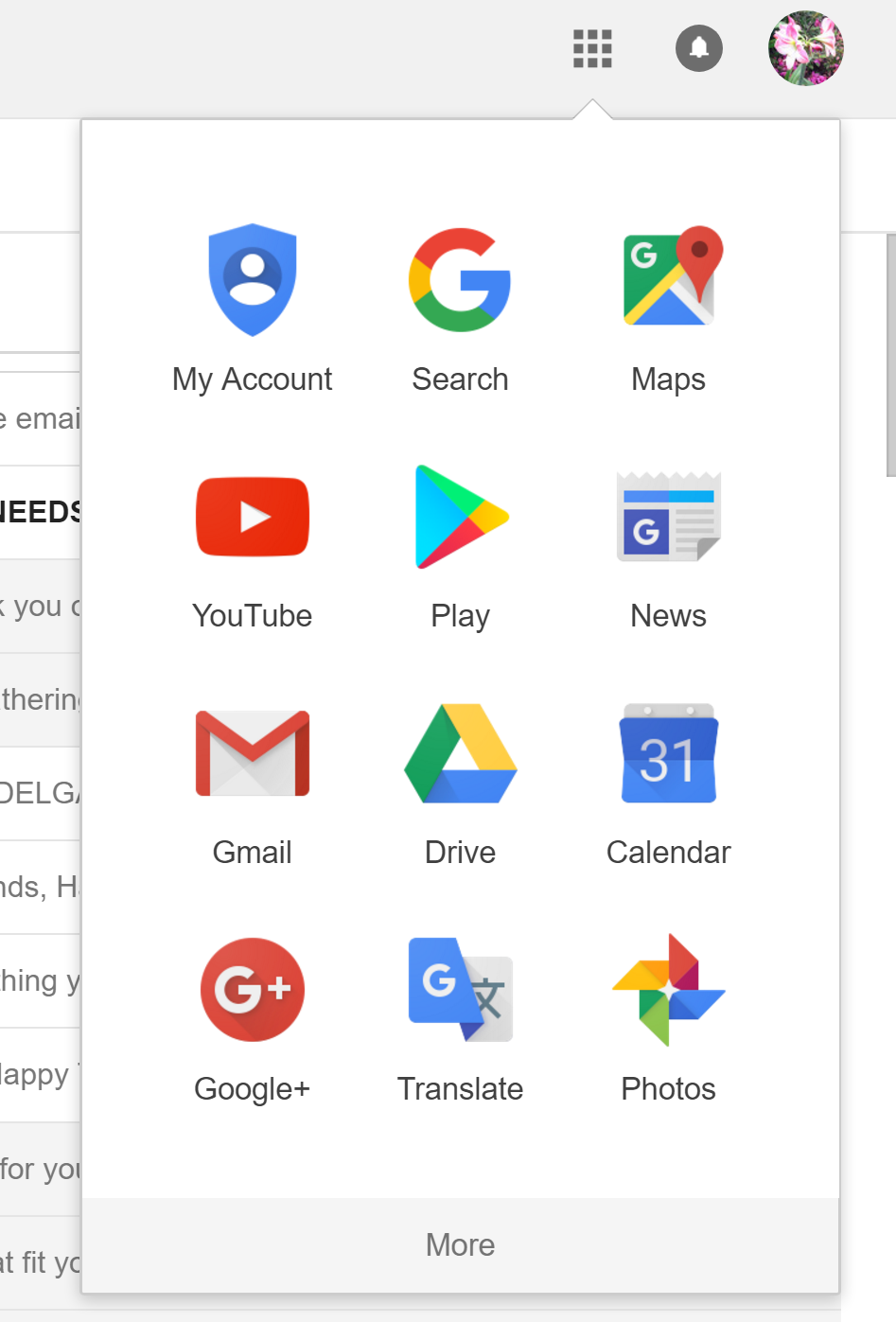The image is a screenshot featuring a user interface with several distinctive elements. At the top, there is a light gray header containing various icons. On the left side of this header, there are three black squares arranged in a row of three. To the right of these squares is a black circle with a bell icon inside, suggesting notifications. Further right, there is a profile picture that appears to be a flower.

In the center of the image, a white menu box is opened, emanating from the nine-square grid icon. This menu displays twelve different icons organized in a 3x4 grid. Below these icons, there is a "More" button, indicating additional options available upon clicking.

The icons in the first column, from top to bottom, are labeled: My Account, YouTube, Gmail, Google Plus. The middle column icons are labeled: Search, Play, Drive, Translate. The right column icons include: Maps, News, Calendar, Photos.

Behind this menu box, there is some obscured text partially visible, with legible words including "happy" and "for you."